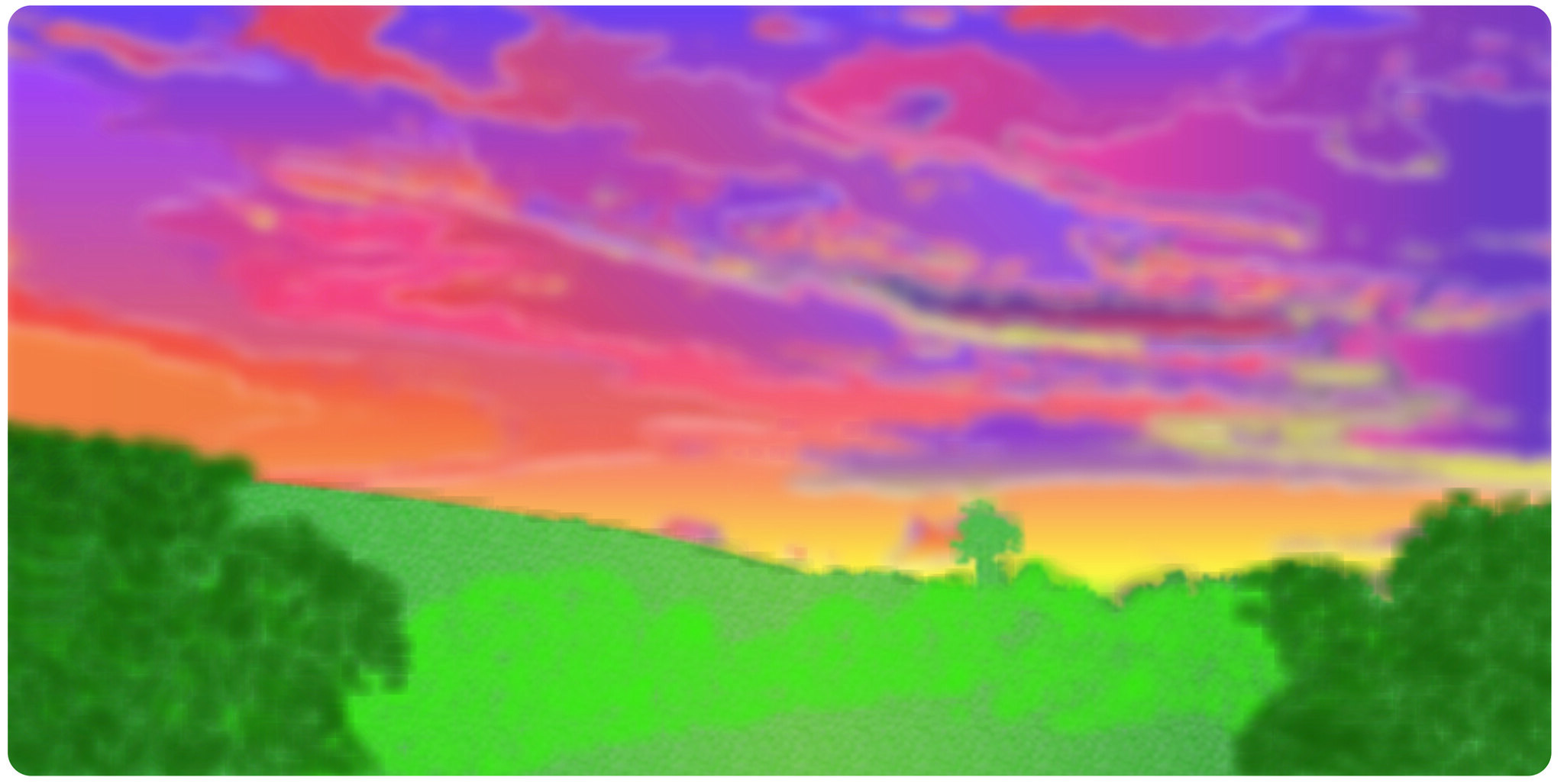The image appears to be a somewhat pixelated and out-of-focus digital artwork, reminiscent of a scene from a video game or computer-drawn illustration. The landscape features a simplified green backdrop with varying shades of light and dark green, representing grasses and bushes. A solitary light green tree stands prominently on the horizon, positioned on a hill. The sky above the landscape is intensely vibrant and dramatic, filled with an over-the-top display of colors. The sunset sky transitions from bright neon oranges and yellows at the horizon, through fuchsia, purples, and pinks, intermixed with mottled patches of white. This kaleidoscope of colors creates an impressionistic and blown-out effect, rendering the scene highly dramatic and somewhat abstract, with swirling clouds and indistinct forms merging together.